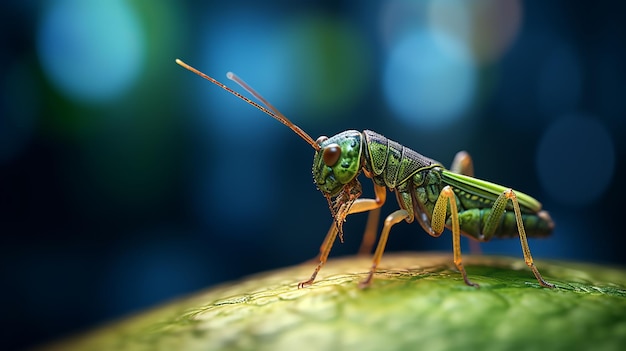The photograph is an exceptionally detailed, high-quality close-up of a metallic green grasshopper, captured with professional clarity. The insect stands on a heavily veined green and yellow leaf, oriented with its back towards the right and its eyes facing left. The grasshopper's head, thorax, and back are a striking metallic green, adorned with black spots and stripes. It has large, bulbous brown eyes and two long brown antennae extending from its forehead. Its legs exhibit a mix of yellowish-brown hues with various black and green spots, highlighting the insect's intricate texture. The photograph's background is intentionally blurred, showcasing a predominantly blue hue with subtle green tints, which contrasts sharply with the sharp focus on the grasshopper, enhancing its prominence in the image.